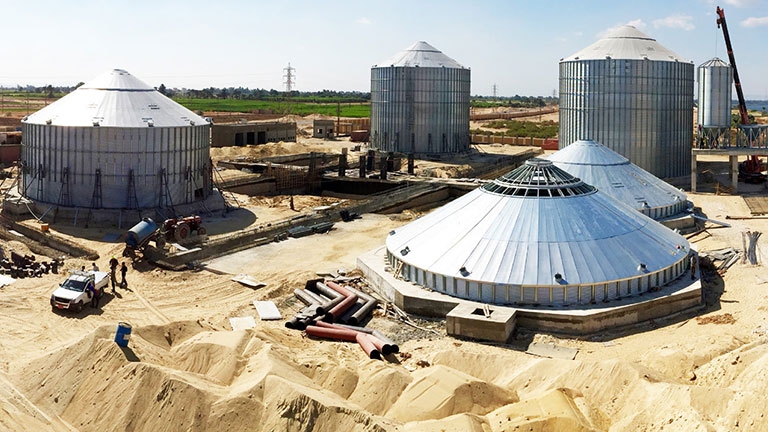The aerial photograph depicts a large agricultural or storage facility under construction in a mostly dirt-covered square area surrounded by green fields. Central to the image are three tall, metal silos with triangular roofs, and two smaller, triangular-roofed buildings positioned to the right front, one behind the other. Scattered around the area are multiple piles of dirt and red and black pipes. Towards the bottom-left corner, a white pickup truck is encircled by several workers, emphasizing ongoing construction activity. An imposing crane stands in the far right background, seemingly lifting one of the silo structures. The dirt area is crisscrossed with roads and bordered by grassy terrain, dotted with utility poles and telephone lines, highlighting the complex nature of the site.